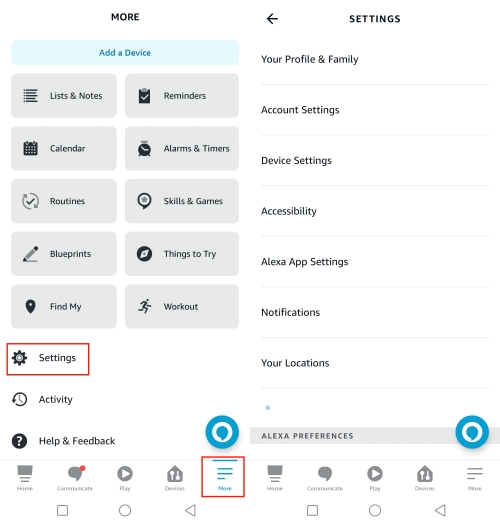The image depicts an Alexa settings page. In the top left corner, there's a "More" section, while the top right is labeled "Settings" with an arrow pointing forward.

Under the "More" section, there's a prominent blue rectangular button with blue font labeled "Add a Device." Below this are ten clickable gray boxes, arranged in two rows of five each. The first row includes:
1. Lists and Notes - with an accompanying icon.
2. Reminders - with an accompanying icon.
3. Calendar - with an accompanying icon.
4. Alarms and Timers - with an accompanying icon.
5. Routines - with an accompanying icon.

The second row includes:
1. Skills and Games - with an accompanying icon.
2. Blueprints - with an accompanying icon.
3. Things to Try - with an accompanying icon.
4. Find My - with an accompanying icon.
5. Workout - with an accompanying icon.

Below these boxes, there is a selected "Settings" button outlined in red, followed by "Activity" and "Help and Feedback" buttons, each accompanied by their respective icons.

On the right side of the page under "Settings," the following options are listed:
1. Your Profile and Family
2. Account Settings
3. Device Settings
4. Accessibility
5. Alexa App Settings
6. Notifications
7. Your Locations

Beneath these, there's a gray search bar labeled "Alexa Preferences."

At the bottom of the screen, there are icons with text underneath stating their functions. They read:
1. Home
2. Conversations
3. Play
4. [Illegible text]
5. More - highlighted with a red square and a chat icon above it.

On the bottom line of the interface, there are symbols depicting:
- A square
- A circle
- A left arrow
- A space bar
- A square
- A circle
- A left arrow

The overall layout is focused on organization, making different Alexa settings and tools easily accessible at a glance.